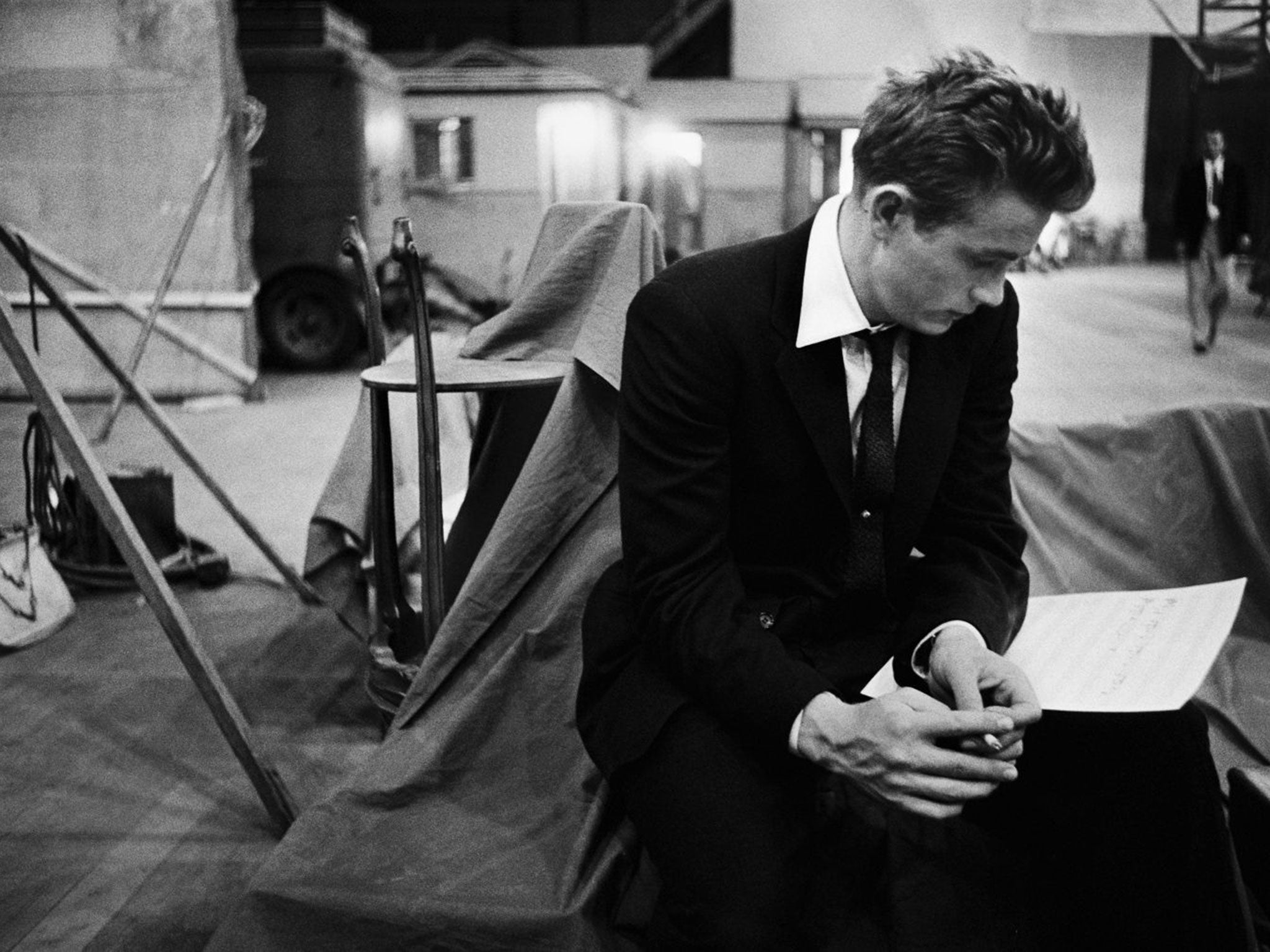This evocative black-and-white photograph, taken by Dennis Stock in 1955, features the iconic actor James Dean. Dean, with his slick, short hairstyle, is seated amidst what appears to be a film lot, possibly outdoors. He holds a cigarette in one hand, intently gazing down at what may be a script or musical score. Dressed in a dark sport coat, a narrow dark tie, and a white sport shirt, he sits on tarps draped over props next to an easel stand. In the blurry background, a man in a suit and tie walks past, and faintly visible are a line of trailers or mobile homes, likely used by actors or crew members. Further details include a vehicle tire, possibly belonging to a van, and large, movable concrete walls that suggest a dynamic Hollywood set.